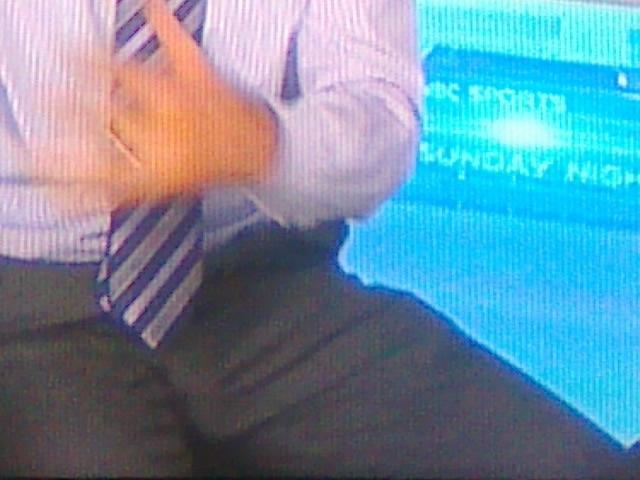The photograph is a close-up of a white male in a sitting position, showing mainly his midsection. He is wearing a white dress shirt with pinstripes and a diagonal striped tie in blue and silver. His dark suit trousers contrast against the shirt. His right hand, visibly blurred due to motion, is positioned in front of his stomach area. The background features a greenish display screen with running text, partially readable as "NBC Sports" and "Sunday Night". The image emphasizes the man's attire and the partially visible text on the screen behind him.